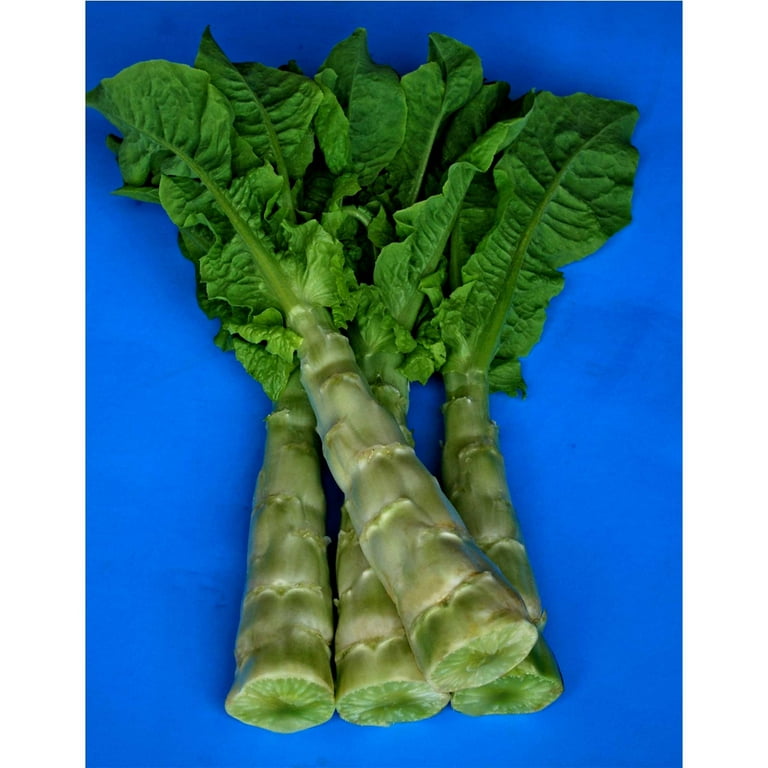This image captures four large, leafy green stalks that strongly resemble asparagus at the base, but with dark green, elongated, leafy tops. The stalks, thick and ridged, are distinctly cut at the bottom, revealing a kiwi-green interior with visible grain. Positioned against a vivid blue background, possibly a table, the brilliant contrast enhances the natural beauty of the plants. While their exact identity remains uncertain, they may be some type of food-related plant, evoking comparisons to vegetables like spinach or bok choy. The variation in green hues and the simple but striking composition make it a captivating photograph of an unusual, possibly edible, plant.